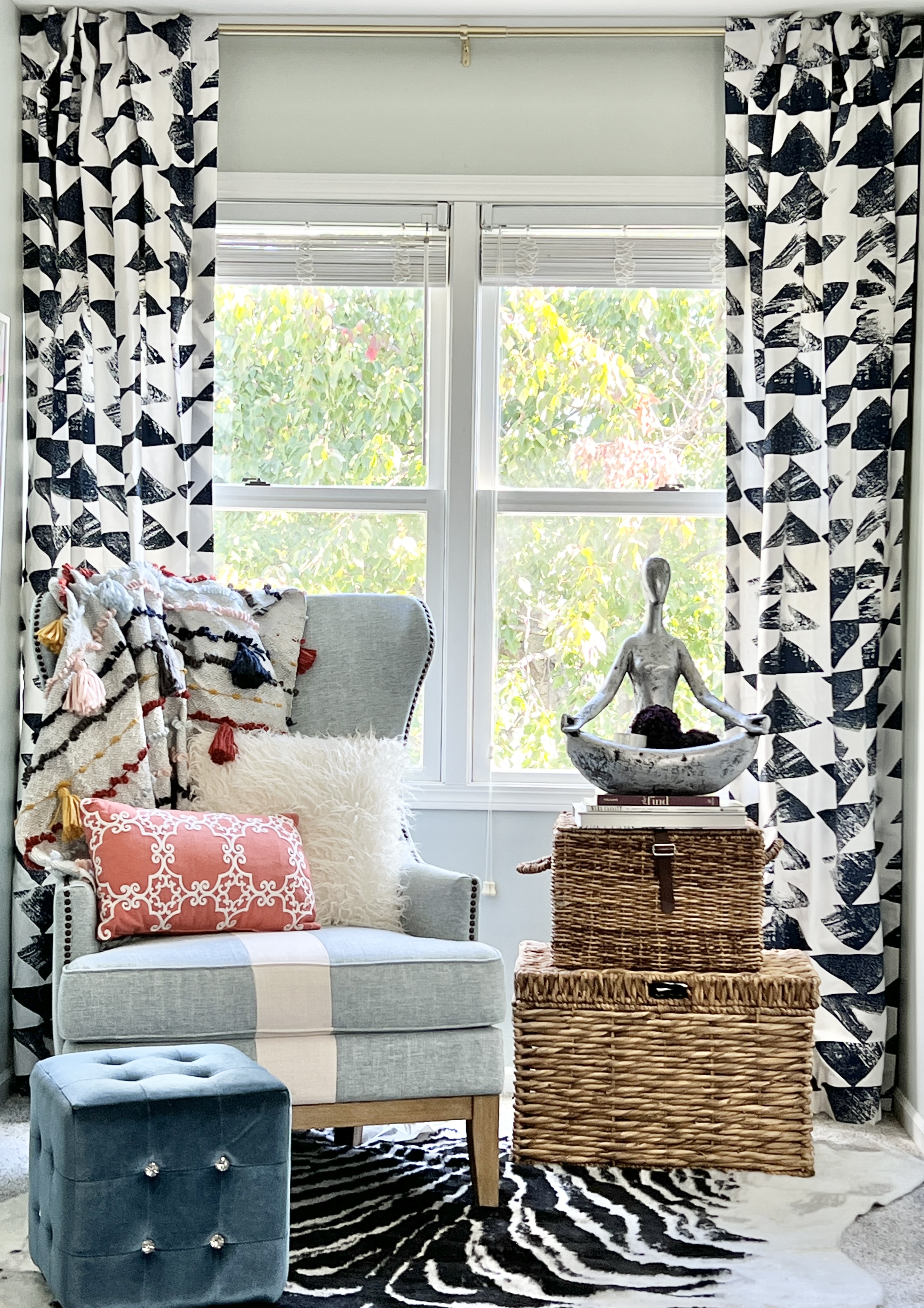This detailed photograph captures a cozy living room scene framed by a large, dual-panel window that offers a view of greenery and sunlight outside. The window is bordered by tall, black-and-white geometric patterned curtains featuring a series of faded black triangles. A plush, bluish-gray chair, positioned slightly to the left in front of the window, is adorned with a fluffy white pillow and a smaller, ornate pillow decorated in pink tones. A colorful, tasseled blanket in shades of blue, red, and yellow drapes over the back of the chair, adding a vibrant touch. In front of the chair sits a teal velvet cube footstool, tufted with four silver buttons, resembling a large die. To the right of this cozy setup are two woven, twined wooden boxes, with the smaller one stacked on top of the larger. These boxes serve as a base for a serene, artistic silver statue portraying a cross-legged, meditating figure. The floor is partially covered by a zebra-patterned rug, which adds an additional layer of texture and warmth to the room.